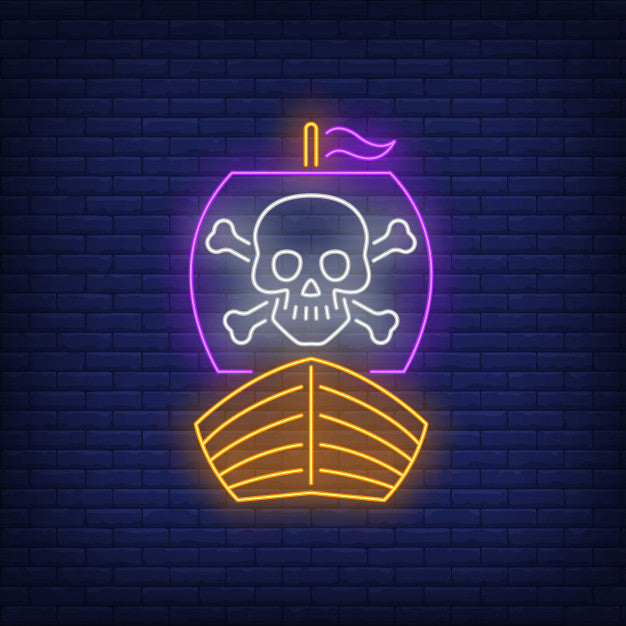This close-up photograph captures a neon sign against a dark blue brick wall, illuminated in the nighttime. At the forefront of the image is an orange neon pirate ship. The ship's bow, outlined in vivid orange with detailed outlines of the wooden slats, faces directly towards the viewer. Rising above the ship is a large sail dominated by a Jolly Roger symbol. The Jolly Roger consists of a white skull with distinct triangular eye holes, a nasal cavity, and a mouth denoted by four lines, while edges of the crossed bones forming an 'X' are visible behind the skull. This emblem is enclosed in a purple neon rounded square. Extending from the top of the sail is an orange mast, which supports a small, triangular flag outlined in purple neon, seemingly waving. The dark blue brick backdrop accentuates the bright neon colors, showcasing the dynamic and vivid imagery of the scene.